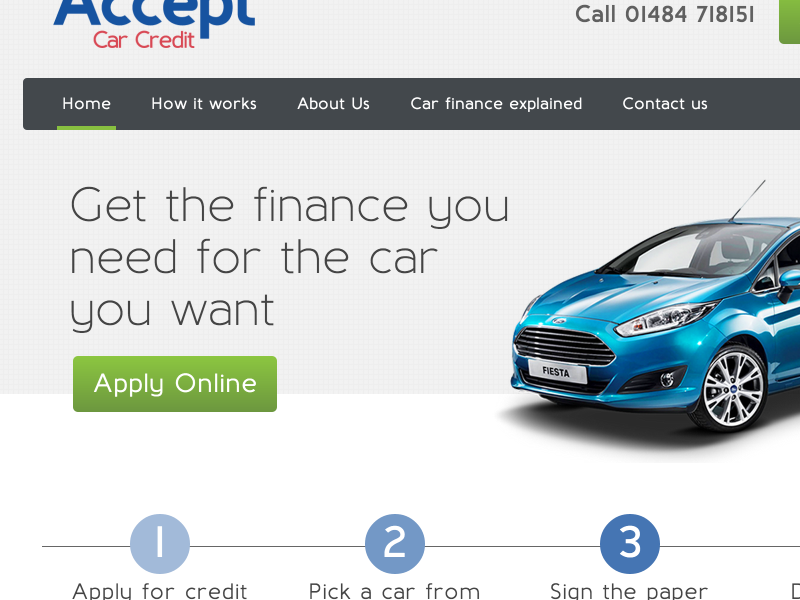The image depicts a promotional website for a car dealership, emphasizing their car credit services. The header features the phrase "Accept Car Credit" in a cut-off manner, with "Accept" in navy blue and "Car Credit" in red, partially obscured by the website's design.

A prominent red strip across the top of the webpage lists navigation options: "Home," "How It Works," "About Us," "Car Finance Explained," and "Contact Us." The "Home" option is underlined in lime green, indicating the current page. Below the header, the text "Get the finance you need for the car you want" encourages potential customers to apply for financing online.

A green box labeled "Apply Online" is prominently displayed, emphasizing the ease of the application process. The main visual on the page is an image of a blue car, possibly a Ford Fiesta, with a visible license plate.

Towards the bottom of the webpage, a step-by-step guide illustrates the process for obtaining car credit, connected by a sequential line:
1. **Apply for Credit** 
2. **Pick a Car**
3. **Sign the Paperwork**

Each step is represented by a blue circle with large, easy-to-read numbers inside.

For further assistance, the website provides a contact number, 01484 718151, and offers the option to reach out via email.